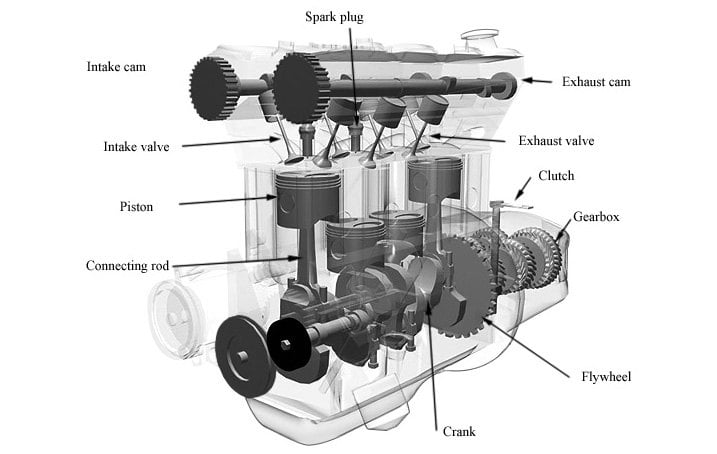The image is a highly detailed, black-and-white diagram of a car's engine, resembling a computer-generated rendering. This grayscale visualization features a four-piston engine with a single crankshaft, clearly depicting each part through labeled black arrows that point to various components. The diagram includes the spark plug, intake valve, piston, connecting rod, and two cams responsible for valve motion. Also shown are the exhaust valves, which are simplified as tubes, along with the intake cam, exhaust cam, and a series of gears. Towards the back of the engine, the clutch, gearbox, and a flywheel are prominently displayed. The engine crankcase is rendered transparent, providing an unobstructed view of the internal mechanisms. The entire setup is meticulously labeled in black text, with notable parts such as the crank and the valve mechanisms situated against a predominantly white background, enhancing the stark contrast typical of such technical illustrations.